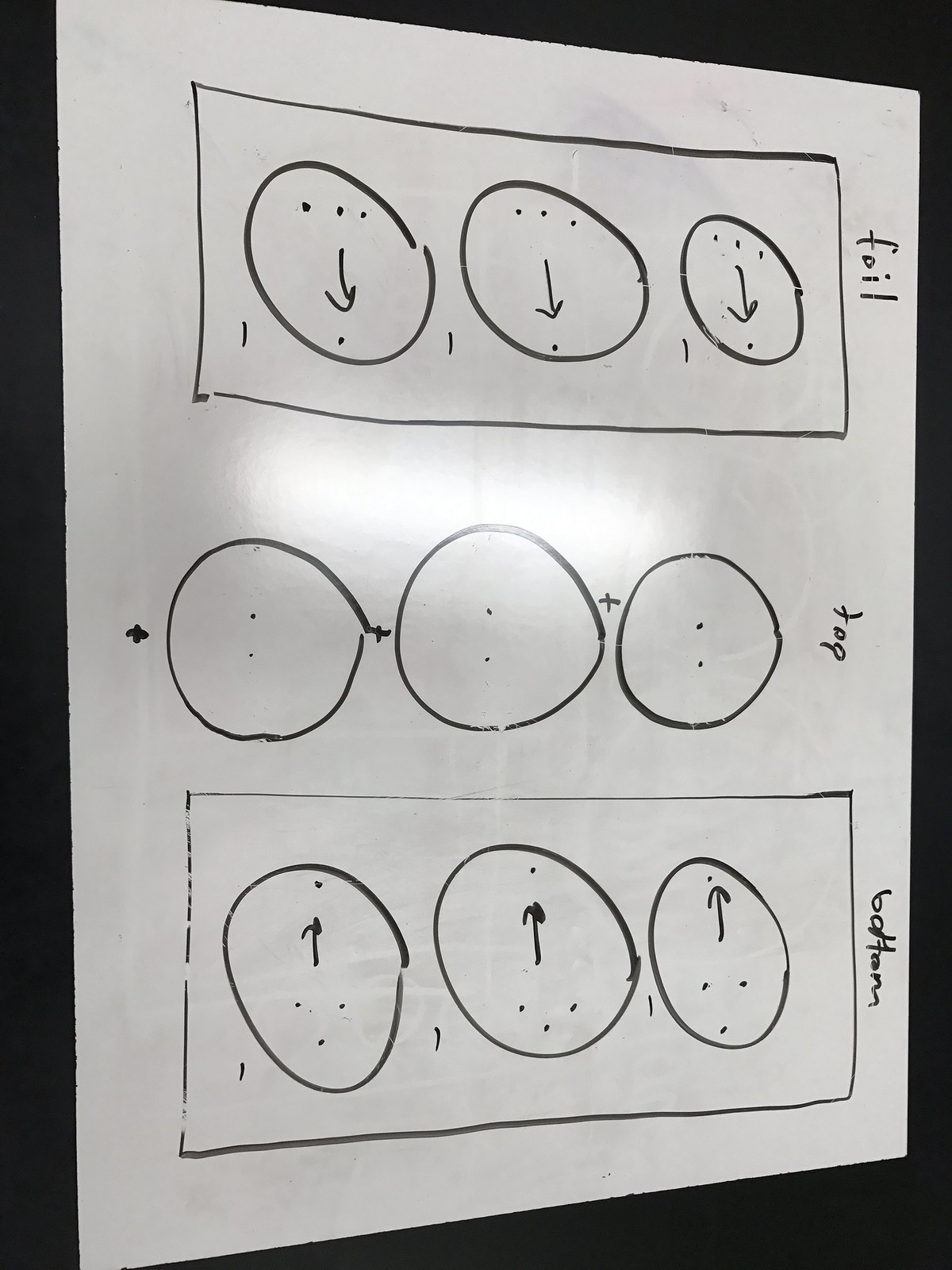This photograph displays a diagram composed of nine circles arranged within three distinct rectangular sections. The top rectangle is labeled "Foil" and features individual dots inside each circle, with arrows pointing from groups of three dots at the tops of the circles to the single dots at the bottoms. The bottom rectangle is labeled "Bottom" and showcases dots in a triangular configuration within each circle, with arrows pointing upward towards single dots. The central rectangle is labeled "Top" and contains pairs of dots within each circle. Additional elements include a plus sign in the center and various arrows connecting dots within the circles, suggesting movement or changes. 

The overall layout and detailed annotations, drawn in black Sharpie on a white sheet of paper placed against a black background, hint towards a scientific context. The diagram likely represents a plan for managing or observing changes on culture plates, possibly in microbiological research involving agar plates. The arrows and labeling could indicate procedures for inoculating, monitoring, or transferring microbial colonies within petri dishes.